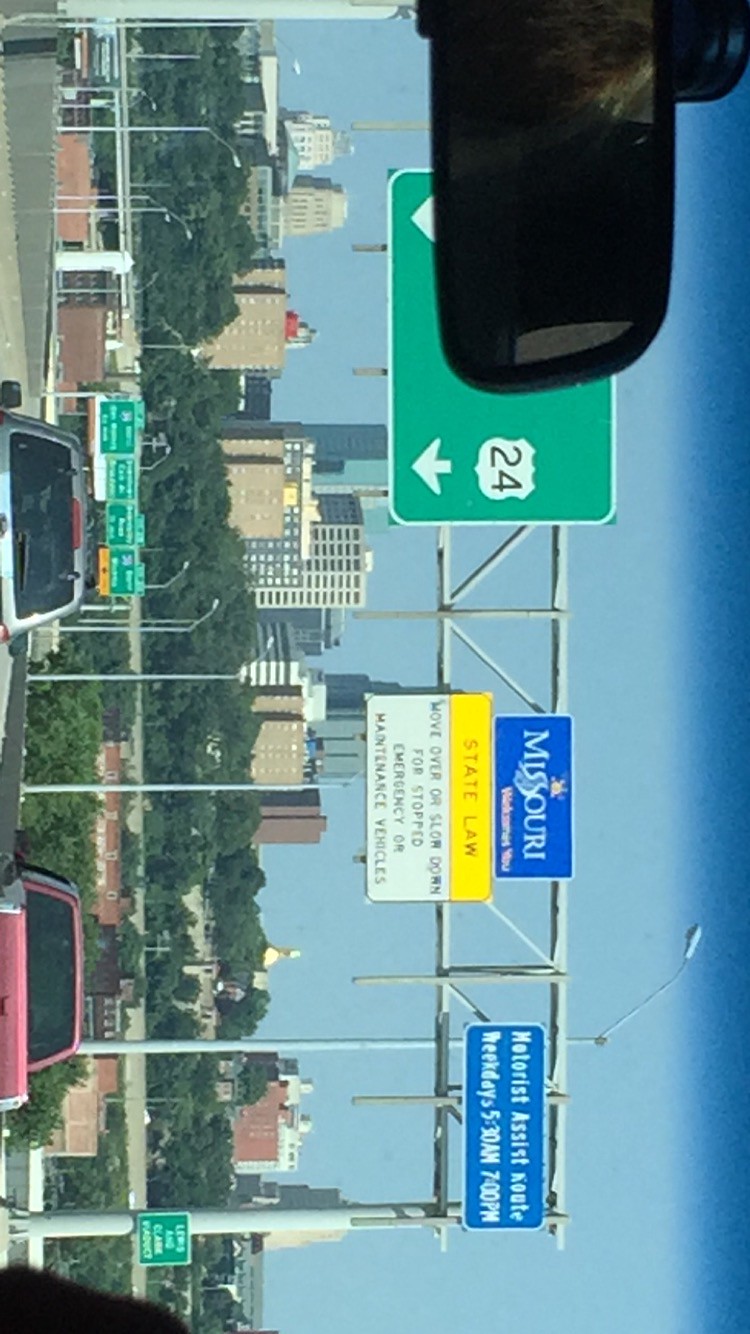The image appears to be taken inside a car, which has been rotated 90 degrees to the right. In the foreground, the rearview mirror captures a blurry reflection, possibly of a dog or someone's hair, suggesting the presence of either a pet or a passenger. The highway scene outside is dotted with several signs, including a prominent blue one that reads "Missouri" and "State Law," although the smaller text beneath it is indistinguishable. The road is moderately trafficked with a variety of vehicles, including a noticeable pink truck and a light blue truck or minivan, enhancing the sense of journeying through a busy interstate.